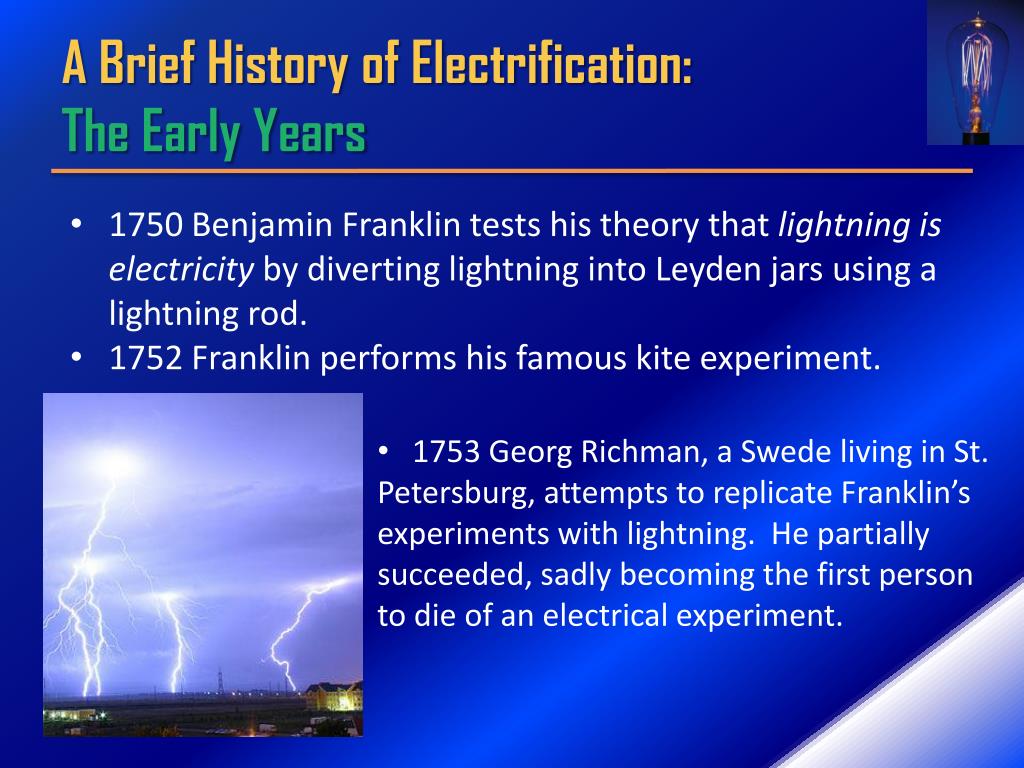The PowerPoint presentation slide titled "A Brief History of Electrification: The Early Years" vividly describes early experiments with electricity. The yellow headline introduces the topic, while a small light bulb icon adorns the top right corner. Beneath the title, the slide is rich in text information, structured with three key bullet points:

1. In 1750, Benjamin Franklin tests his theory that lightning is electricity by diverting lightning into Leyden jars using a lightning rod.
2. In 1752, Franklin performs his famous kite experiment.
3. In 1753, George Richmond, a Swede living in St. Petersburg, attempts to replicate Franklin's lightning experiments. He partially succeeds but tragically becomes the first person to die from an electrical experiment.

The background of the slide is predominantly blue, fading into white towards the lower right corner. Visually enhancing the slide is a larger image in the bottom left quadrant, depicting multiple lightning bolts striking the ground from a brown landmass, emphasizing the theme of electricity.